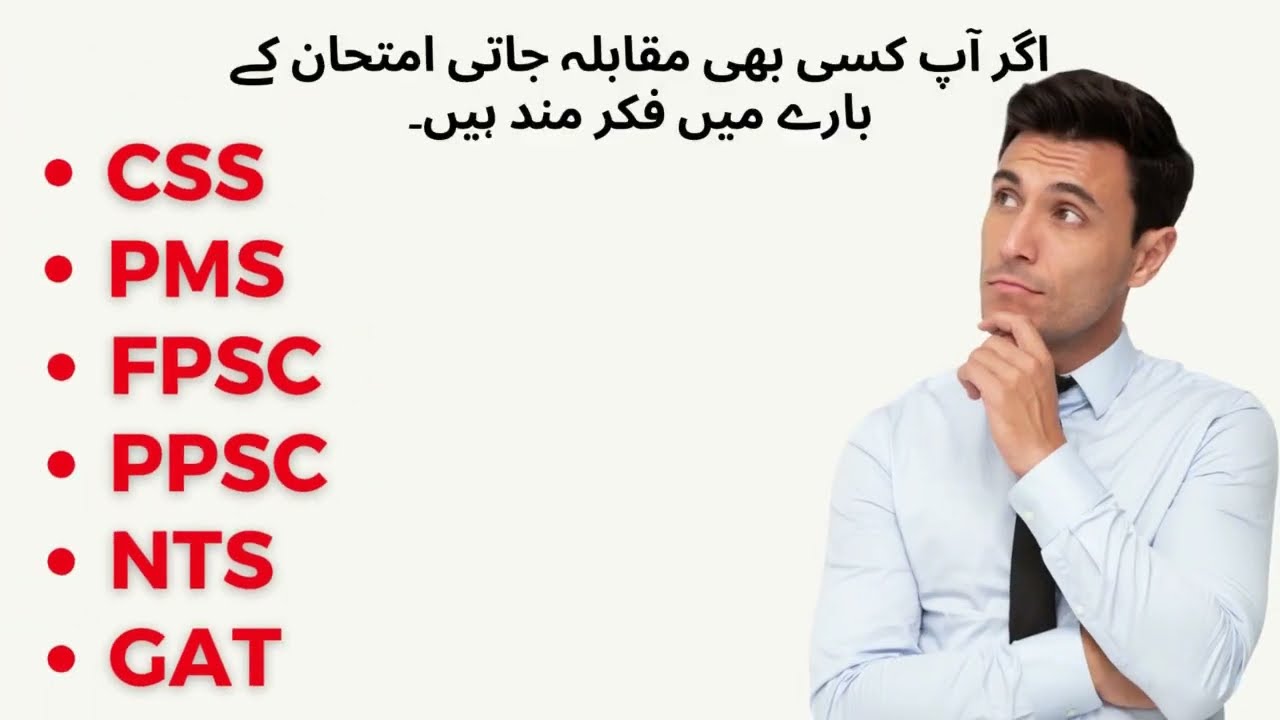The image features a young man positioned to the right, with dark hair, wearing a white button-down shirt and a black tie. He stands in a contemplative pose, his left hand thoughtfully touching his chin, while his right arm is folded under his left elbow. His gaze is directed upwards, toward the top of the slide. Centered at the top of the slide is text in a foreign script, possibly Arabic, in black font. On the left side of the image, there is a vertical list of acronyms in red letters, each preceded by a bullet point. The acronyms are CSS, PMS, FPSC, PPSC, NTS, and GAT.